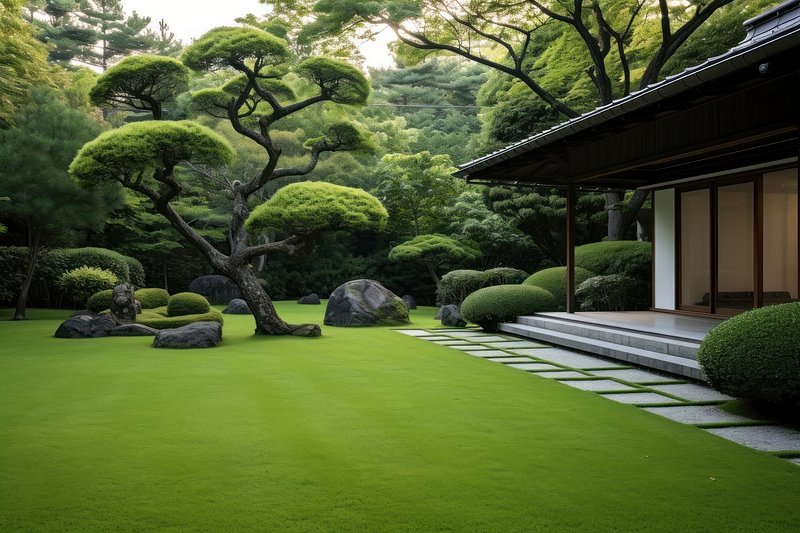The image showcases an immaculate, Japanese-style garden that is almost surreal in its precise and detailed composition. The foreground is dominated by a lush, vivid green lawn, which may appear artificial due to its pristine condition. This area leads the eye to a traditional Japanese-inspired structure on the right, featuring a large black awning and a stone porch, accessed by a set of stone steps. Beneath the porch are three expansive glass panes set into white walls, providing a glimpse into the modern property within. Adjacent to the porch and partially cut off by the frame is a round bush, adding a touch of greenery to the scene.

In front of this porch, an irregularly arranged path of square and wider stones creates a walkway that seems almost playful yet meticulously placed. Off to the left of the image is a tree with foliage resembling green clouds, suggestively a bonsai tree given its precise pruning. Near the tree is a collection of rocks, with one particularly large rock resembling an animal lying down with its feet outstretched, its form blending naturally into the serene setting.

In the background, which is the busiest part of the garden, another bonsai is prominently centered, flanked by neatly shaped topiary shrubs and towering trees that almost fully obscure the sky, save for a few peeks of bright white at the very top. These trees create a natural, yet almost artificial fence encasing the garden, balancing the scene between the natural and the constructed. The overall composition, with its intricate details and precise layout, lends the garden a slightly surreal, almost AI-generated quality, seamlessly blending traditional elements with a modern aesthetic.